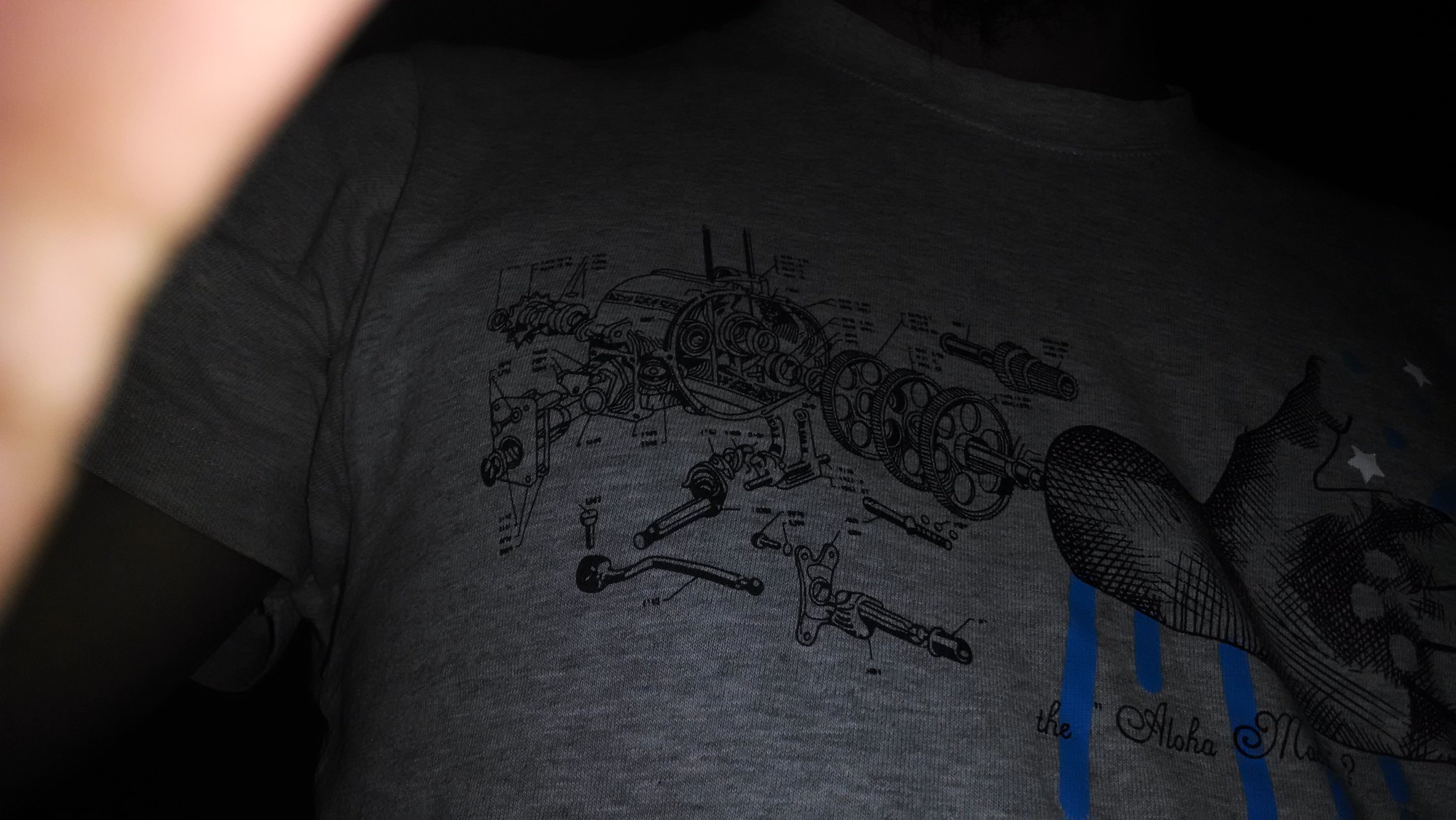This is an extreme close-up color photograph of a person's torso, focusing just below their right shoulder. The image is shrouded in dim lighting, casting much of the scene in shadow and obscuring the person's complexion. However, their attire is discernible: a short-sleeve gray shirt featuring intricate graphics. The design on the shirt resembles a meticulously detailed ink drawing of a machinery schematic. Towards the lower right-hand side of the frame, another drawing appears, possibly depicting a collection of rocks. Adjacent to these illustrations are three vertical stripes, rendered in a vivid blue hue. A small, indecipherable script signature nestles in the same corner, further adding to the shirt's elaborate design.